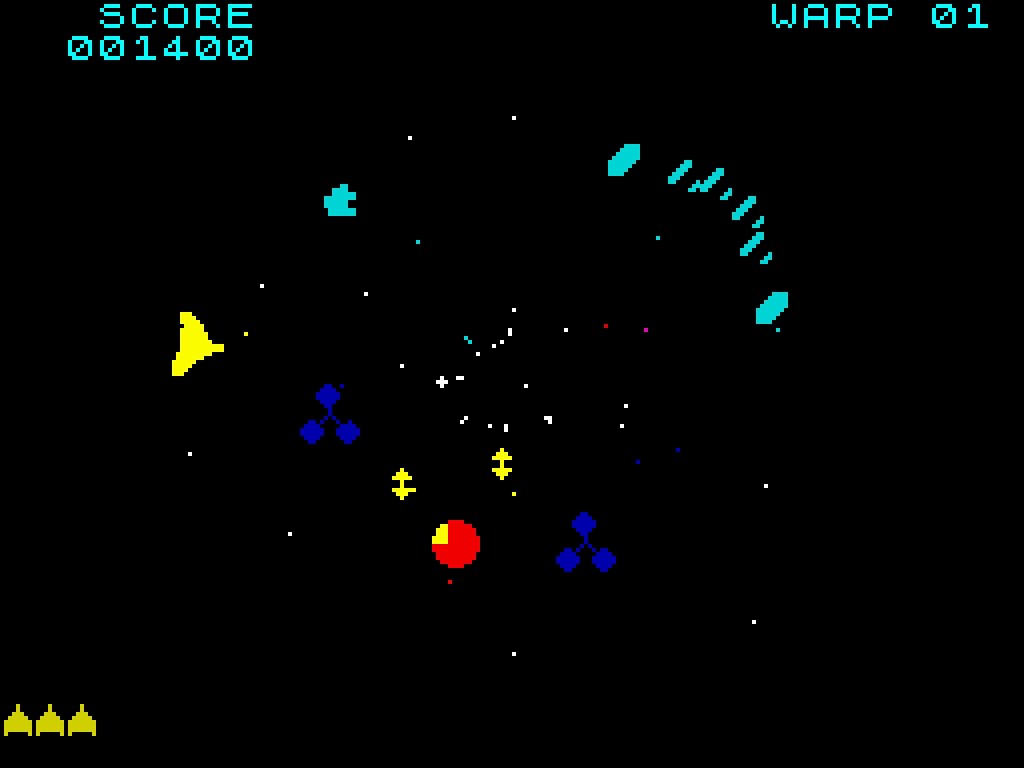The image is a screenshot from a video game, featuring a stark black background adorned with vibrant, colorful lights. Dominating the color palette are hues of red, yellow, blue, light blue, and purple. Prominently displayed at the top edge of the screen are two key indicators: the current score of 1,400, rendered in light blue text, and a warp status labeled "01" also in light blue, positioned to the right.

The player's ship, a distinct yellow arrow-shaped vessel, is situated on the screen, poised for action. To the bottom left of the display, three yellow icons are arrayed, resembling miniatures of the player's ship, likely representing the remaining lives or attempts available.

Facing the player's ship are blue objects that have a hazardous material or emergency sign appearance, characterized by their triangular ends and intersecting lines. Mixed among these are various blue oblong objects, adding to the complexity of the scene. Additionally, there is a prominent red circle with a small yellow sliver missing from it, contributing to the array of visual elements on the screen.